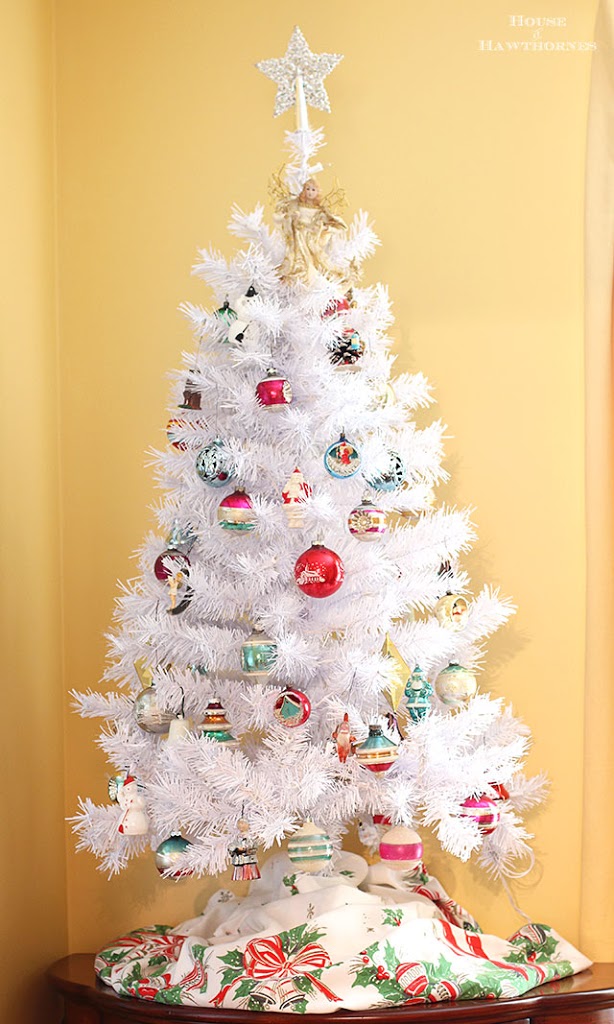This image showcases a small, artificial white Christmas tree set on a dark brown table. The tree's needles are purely white and it's adorned with a variety of colorful ornaments, including pink and green striped baubles, as well as red, blue, and gold shiny metallic bulbs. The tree is topped with a white star and an angel figure in golden robes with long hair, creating an elegant focal point. The tree's stand is covered by a festive tree skirt, predominantly white and decorated with images of green wreaths, red ribbons, silver bells, and green leaves. The background features a warm, dandelion yellow wall, framing the Christmas tree in a cozy, festive ambiance. Additionally, small white text at the top of the image reads "House of Hawthorns."